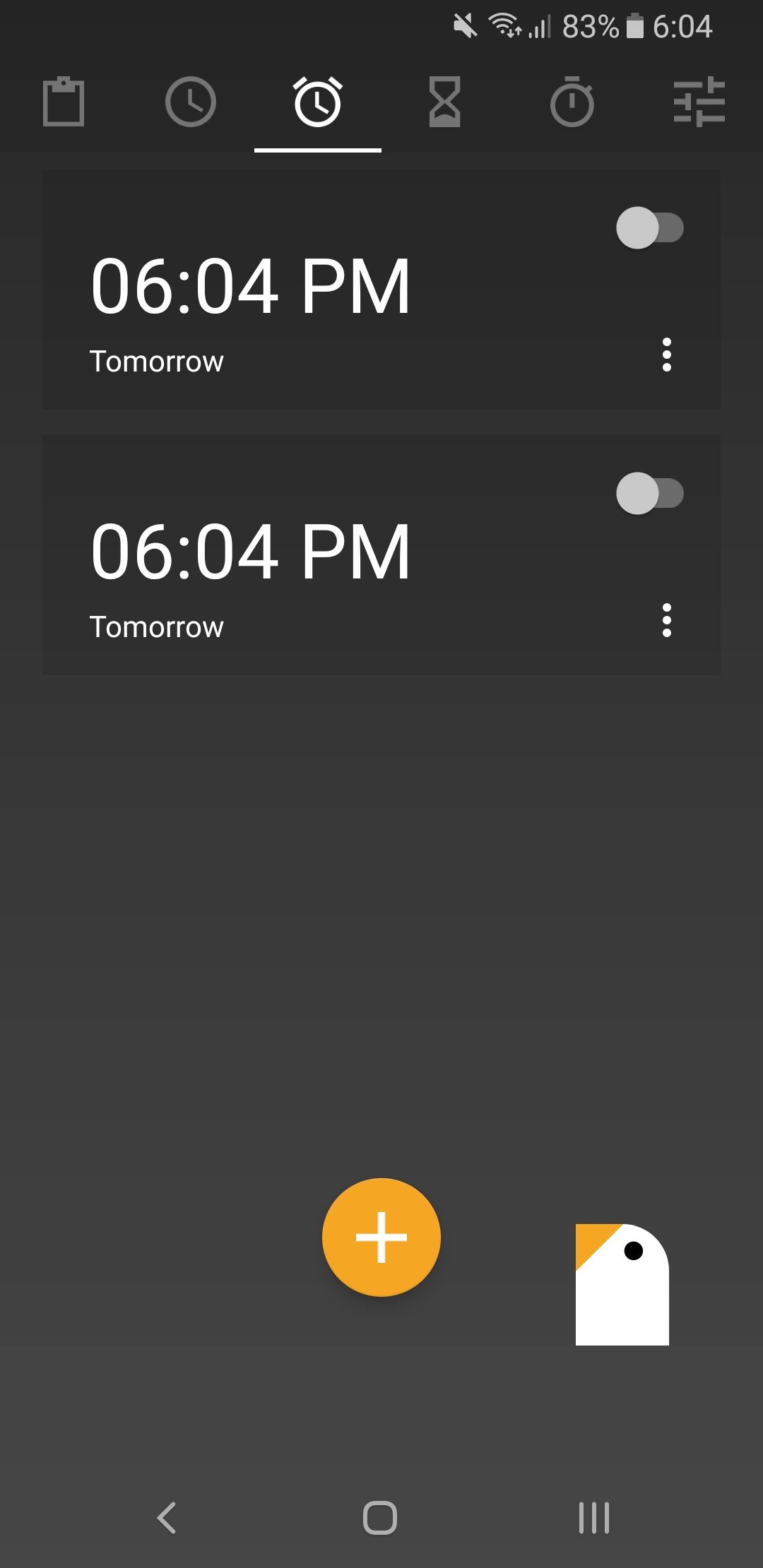This is a detailed screenshot of a mobile device interface, set against a black background and featuring a mixture of gray and white elements for excellent contrast and readability. At the top, icons depict the device's status: a muted speaker symbol (with a slash through it), a Wi-Fi signal resembling a funnel or tornado, signal strength bars, a battery percentage indicator showing 83%, and the current time of 6:04. 

Below these, a series of grayish-white icons are displayed, including a clipboard, a clock, an alarm clock, an hourglass, a stopwatch, and what appear to be switchboard symbols. Each icon is distinctly outlined and clear.

Further down, two alarms are set for 6:04 PM the next day, each indicated by a gray circle and accompanied by three white circles. These elements are both clear and user-friendly, making the settings easy to understand at a glance.

At the bottom of the screen, there are more functional icons: a gold circle with a white plus sign, a white and gold price tag icon with a black dot, and navigation icons in grayish-white—comprising a back arrow, a square, and three horizontal lines.

The image is notable for its high visual quality, bold and user-friendly design, and easy-to-read font. There are no other objects or visual distractions present, making the relevant information stand out clearly with no pixelation or blurring.